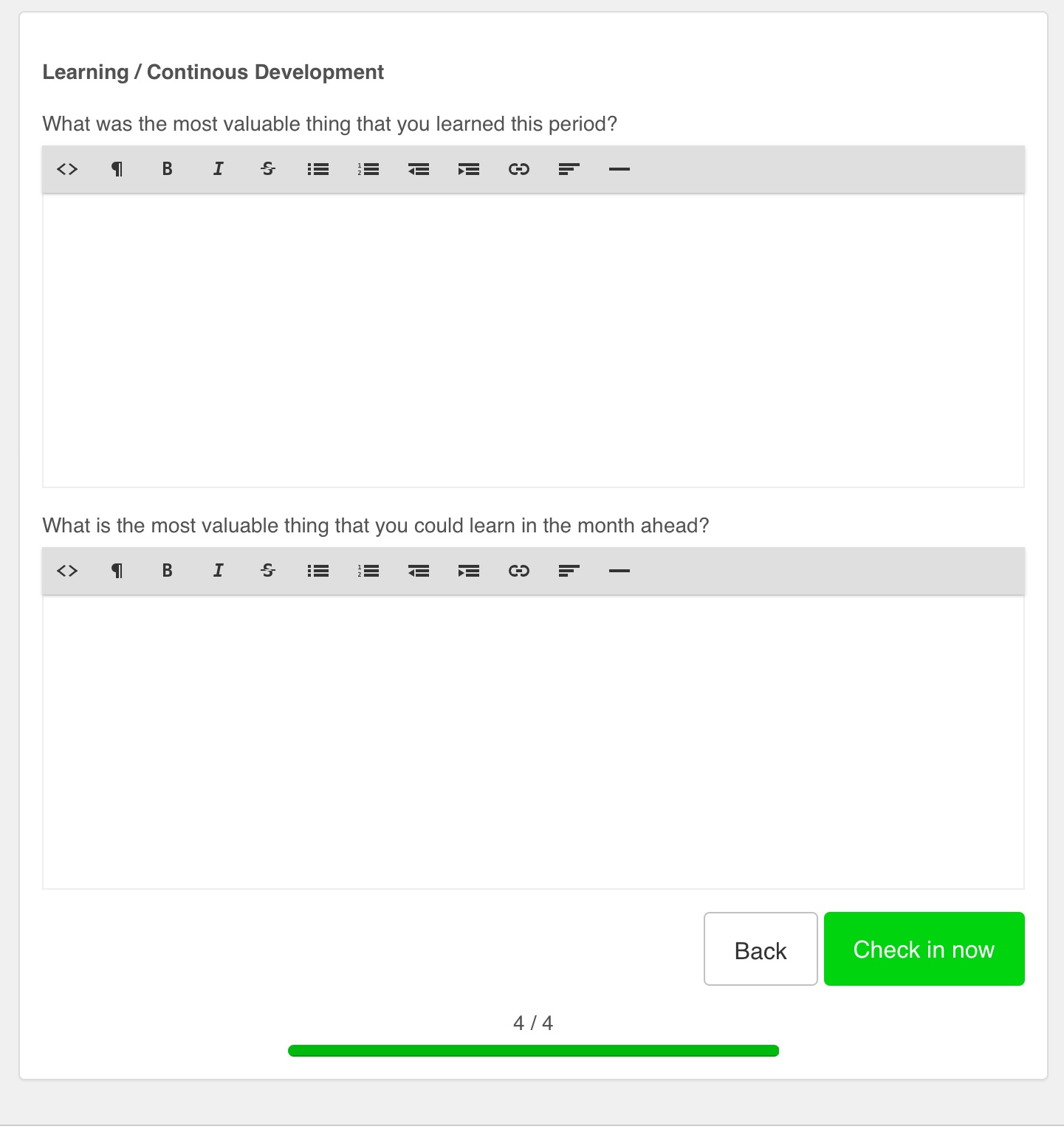The image depicts a screen interface dedicated to gathering user input under the heading "Learning / Continuous Development," which is prominently bolded. Below this heading, two specific questions are displayed, each accompanied by a text box designed for user responses. The first question asks, "What was the most valuable thing that you learned this period?" The text box below it allows users to type their answer and offers various formatting options such as bolding, italicizing, and adjusting text spacing and indentation. 

The second question inquires, "What is the most valuable thing that you could learn in the month ahead?" Similar to the first, it is followed by a text box where users can enter and format their responses as needed. 

Beneath these text boxes, there is a "Back" button that allows users to return to the previous screen. The default option, a green "Check In Now" button, is prominently visible and stands out as one of the few colored elements on the screen. At the very bottom of the image, the text "4 of 4" indicates that this is the final page in a sequence of questions in what appears to be a question wizard.